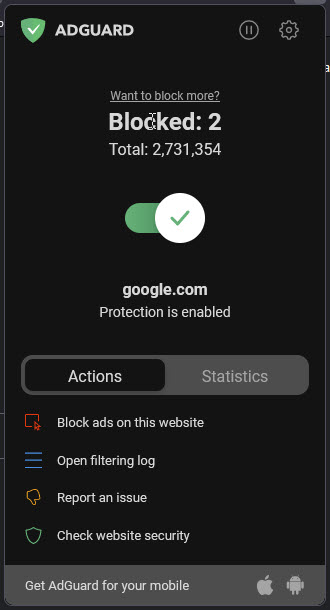The image depicts a user interface for the AdGuard application, presented within a tall, vertically-oriented black box. In the upper left corner, there's a green shield emblem containing a white checkmark. Adjacent to this shield, the brand name "ADGUARD" is displayed in all capital letters.

Toward the center, the phrase "Want to block more?" is written in light gray text and underlined. Just below this question, the word "Blocked" is shown in white text, followed by a colon, and then the number "2." Further below, the word "Total" is similarly followed by a colon, and the figure "2,731,354" is displayed.

Continuing downwards, there's a horizontal green oval next to a white circle that contains a green checkmark, indicating activation. Beneath this section, "google.com" is listed in smaller text. Additionally, it mentions that protection is enabled.

Towards the bottom, two action buttons are visible: "Actions," displayed within a black box, and "Statistics," within a gray box. A red square to the left of these contains the option "Block ads on this website." Below this, three small horizontal blue lines signify "Open filtering log."

Further down, there's an option to "Report an issue." Finally, next to an image on the left showing a green shield, there is a prompt to "Check website security."